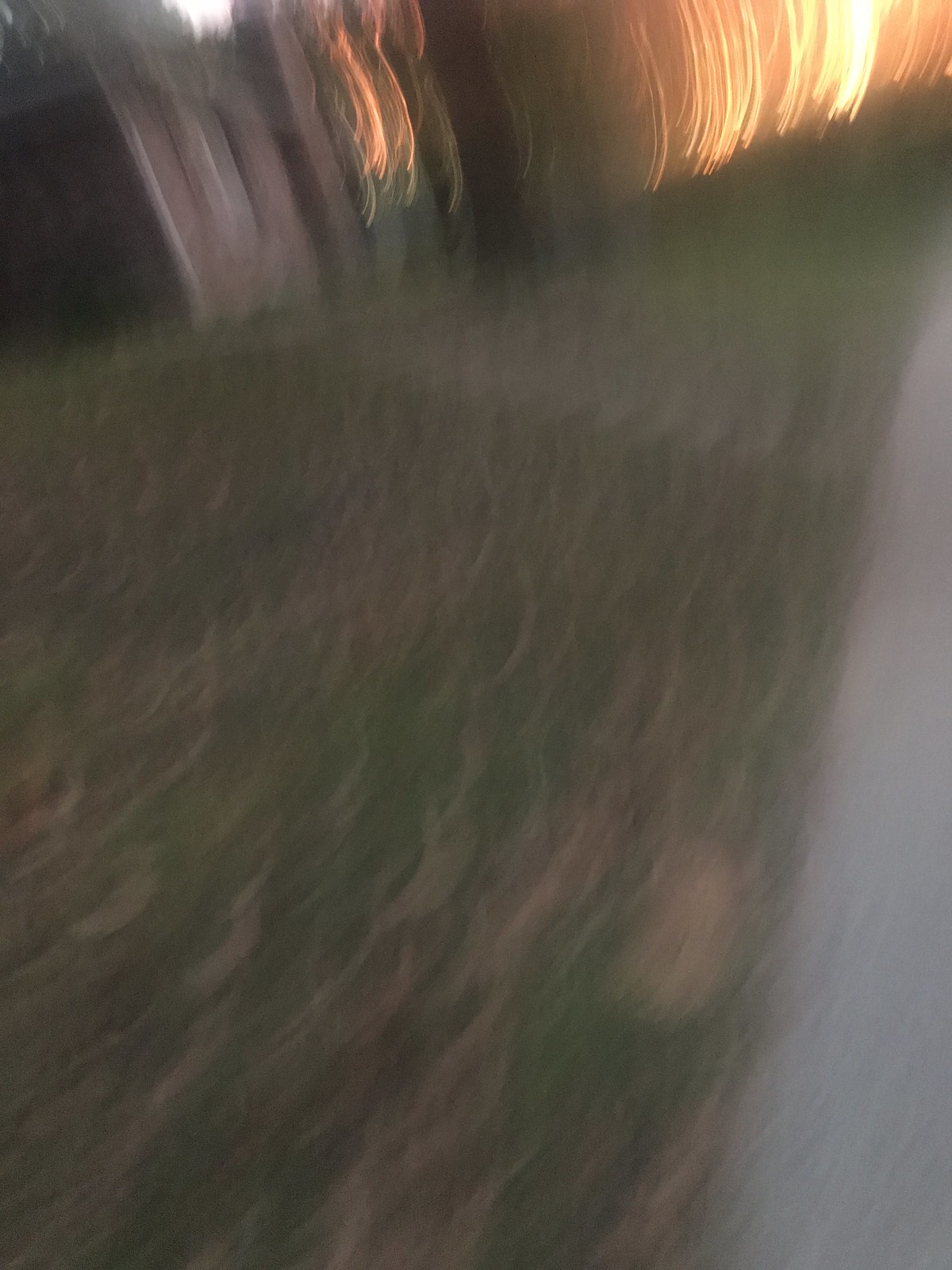The image depicts a sunlit scene resembling a cascading waterfall, where delicate, white, strand-like formations descend gracefully and appear to thicken as they approach the camera. Interspersed among these luminous strands are vibrant green elements, evoking the illusion of movement within a stream. The stream-like feature showcases a mix of green and brown hues, adding depth and texture to the composition. A distinct white border frames the image, creating a striking contrast. The sunlight streams through the strands, highlighting their uniform lengths and enhancing the overall beauty of the scene.